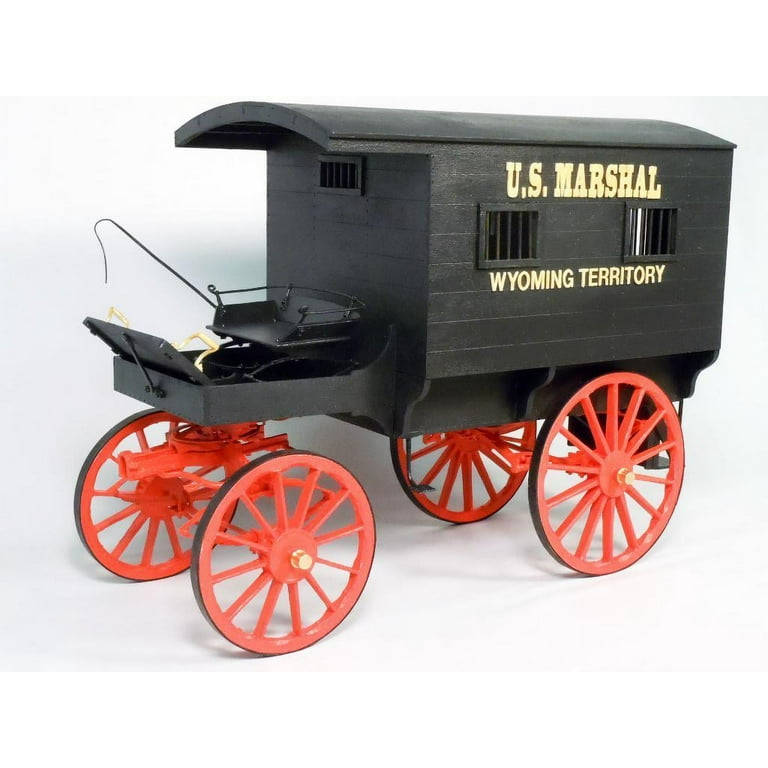The image depicts a detailed replica or toy of a vintage U.S. Marshal stagecoach from the Wyoming Territory. The stagecoach is primarily black with striking red-rimmed wheels, which feature gold spokes. Across its side, the text "U.S. Marshal, Wyoming Territory" is prominently displayed. The windows of the stagecoach are secured with black bars, evoking a sense of it being used perhaps as a prison transport. At the front of the stagecoach, there is a black driver's seat complete with a whip, indicating it would have been used to drive the horses. There also appears to be a step at the very back of the stagecoach for entry and exit. The craftsmanship details make it look like an old-timey piece one might find in a museum.